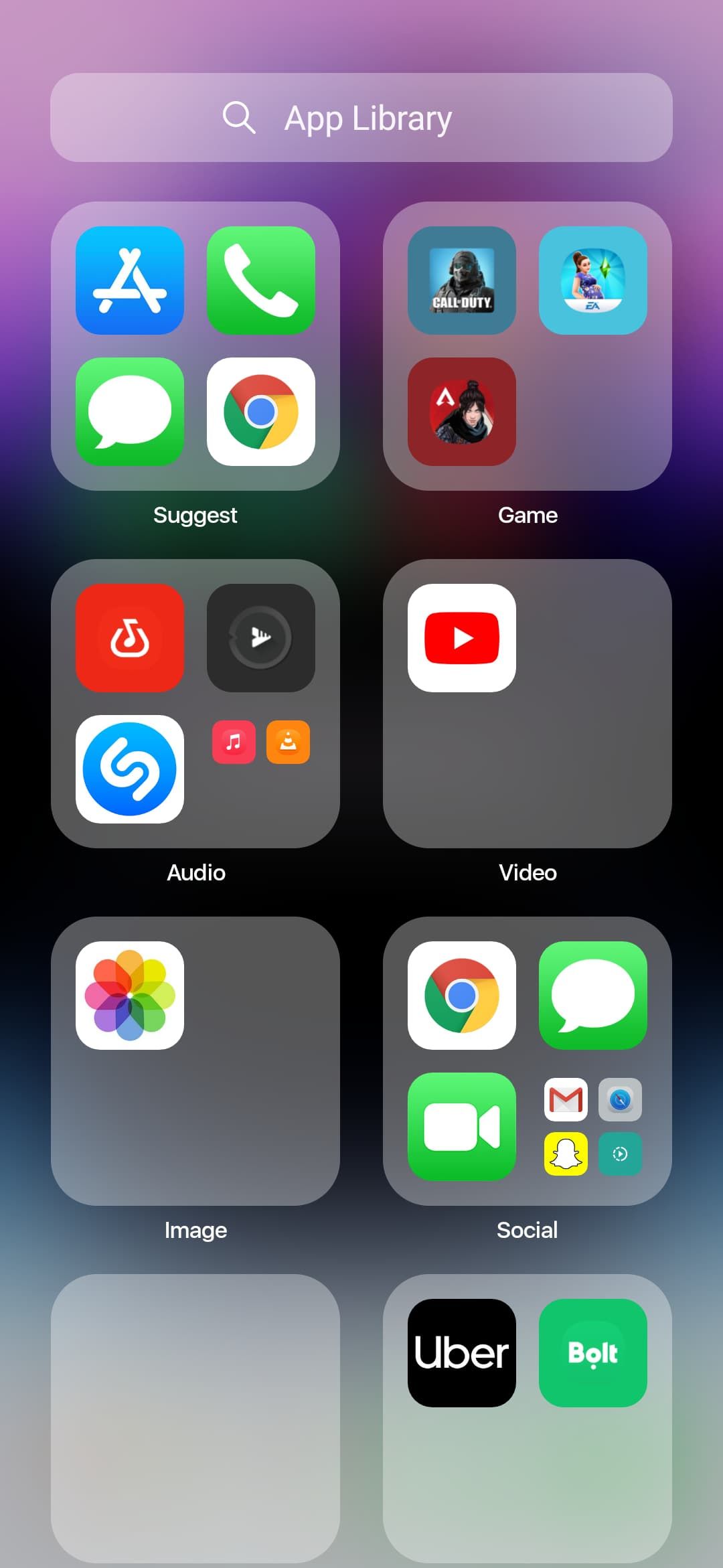This is a screenshot of a smartphone's App Library. At the top, there is a search bar available for finding specific apps within the library. The featured apps and folders include:

1. **Featured Apps**:
    - **Apple Store**: For downloading and purchasing apps.
    - **Telephone**: For making calls.
    - **Texting**: For sending messages.
    - **Google Chrome**: For web browsing.

2. **Categories**:
    - **Games**:
        - **Call of Duty**: Placed prominently in the first slot.
        - **Two other games**: One of them is unrecognized.
    - **Audio**:
        - Three major audio apps are visible, along with two smaller ones.
    - **Video**:
        - **YouTube**: Clearly displayed for video streaming.
    - **Images**:
        - **Google Photos**: Available for managing and viewing images.
    - **Social Media**:
        - **Google Chrome**: Also categorized under social.
        - **Messaging**: For various text and chat communications.
        - **Video Maker**: For creating video content.
        - **Email**: For handling electronic mail.

3. **Notifications**: Likely a button or area for managing notifications and related activities.
4. **Other Apps**:
    - **Uber**: For ride-hailing services.
    - **Bolt**: Another ride-hailing service option.

This user appears to use their phone extensively for communication, media consumption, and various utilities.